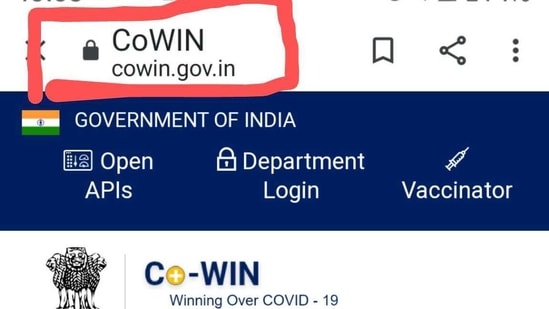This image focuses on the webpage for coen.gov.in, highlighting specific user interface elements. The website address is prominently displayed at the top, with "Coen" outlined in a bold red rectangular marker that partially overlaps the 'X' on the webpage. Adjacent to the address bar are several icons, including a bookmark, a share option, and a menu represented by three vertical dots. 

Underneath the address bar, a blue banner is visible, featuring the Indian flag and the text "Government of India." The banner also includes an icon resembling some type of machinery followed by the words "Open APIs." To the right, there's a lock icon next to "Department Login," and a needle-like icon next to the word "Vaccinator."

The lower section of the image has a predominantly white background. On the left-hand side, there are three lines: the first is horizontal while the other two face opposite directions, one looking left and the other right. A dividing line bisects this segment with the text "Co-WIN," accompanied by a plus and minus sign. The plus sign is notably placed inside a yellow circle.